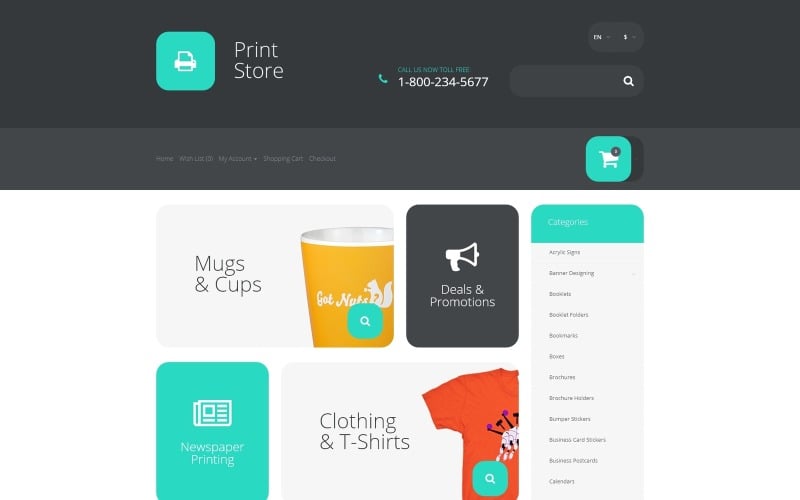Under the heading "Websites," this image is relatively condensed, with various semi-small elements. At the top, it features a fairly large black bar, distinguishing it from thinner bars commonly seen on websites. Within this black bar, there's a teal box displaying a printer icon alongside the text "Print Store." Adjacent to this is the call-to-action "Call us now toll free 800-234-5677," accompanied by a small phone icon indicating that the service is available in English. Additionally, a search bar, complete with a magnifying glass icon, is placed alongside these elements.

Beneath this primary bar is a slightly lighter bar containing white text, though some of the content is illegible. However, it does feature an icon of a shopping cart with what appears to be one item inside.

Below this section, the image transitions to a white area showcasing various categories. The first category, labeled "Mugs and Cups," includes an illustration of a yellow cup with a squirrel design and the text "Got nuts?" Another category, "Newspaper Printing," is listed without an accompanying image. The "Clothing and T-Shirts" category is represented by a fragment of an orange t-shirt. Lastly, the "Deals and Promotions" category is marked by a megaphone icon.